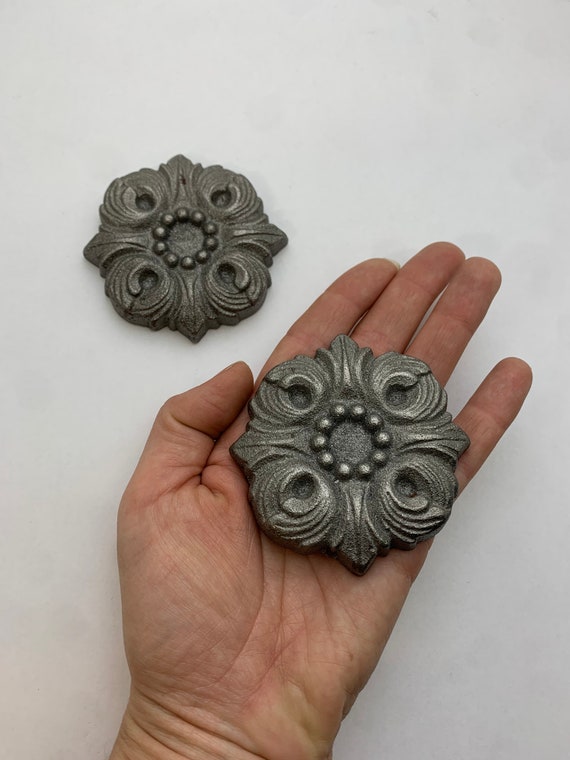The image features a close-up view of a Caucasian person's left hand, palm up, against a stark white table background. The hand, devoid of rings or a watch and with a slightly dark skin tone, holds a dark gray and black medallion-like object. The medallion, intricately designed, has a square base with highlighted corners. Each corner extends into a compass rose-like pattern pointing in the cardinal directions, interspersed with plume-like feather designs. At the center, a circular wreath composed of small round beads or dots is prominently featured. To the upper left of the hand, an identical medallion lies flat on the table. The hand's fingers are straight while the thumb is bent towards the pointer finger, adding to the detailed and focused composition of the photograph, which emphasizes the unique and detailed design of the objects.